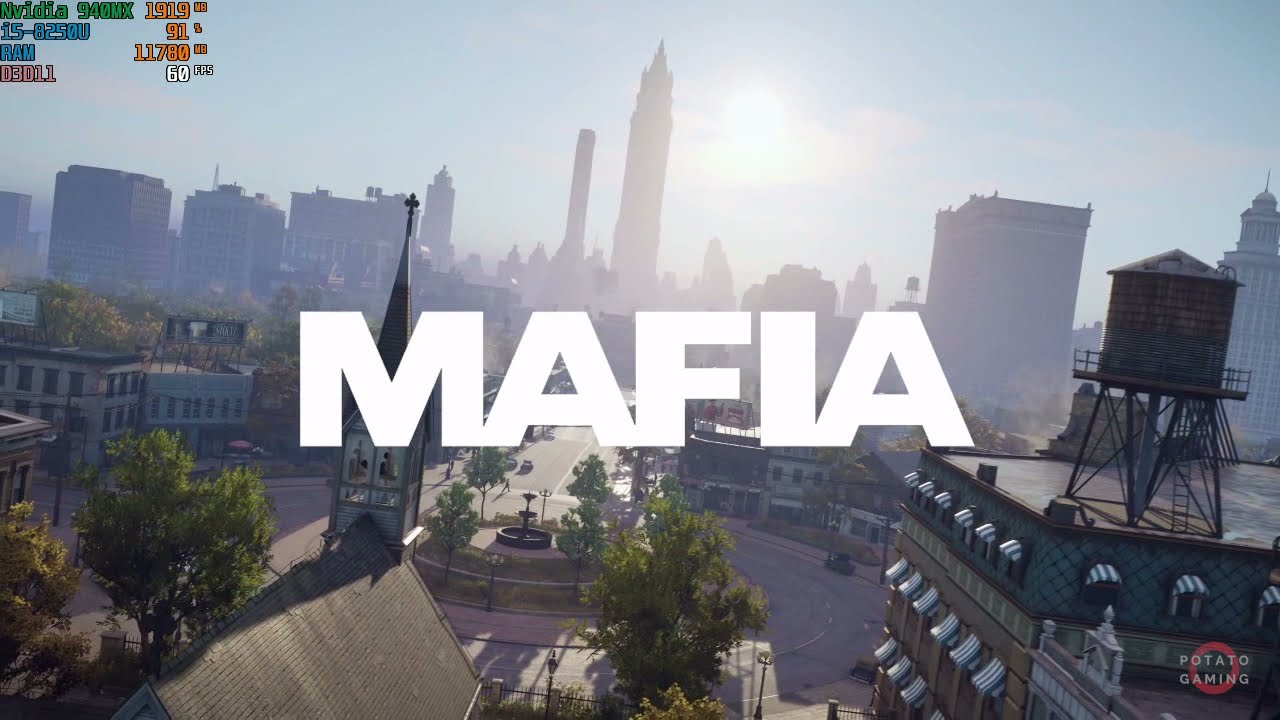In this detailed screenshot from the video game "Mafia," we are presented with a vibrant urban scene. Dominating the center of the image in large, bold white capital letters is the title "MAFIA." The city landscape includes a prominent roundabout surrounded by various buildings, including colonial-style structures and more modern skyscrapers. A well-manicured garden with trees and a fountain enhances the roundabout's center. Below, there is a distinct church with a steeple, and nearby, a rectangular building topped with a small water tower. The upper portion of the image showcases the city's skyline under a hazy blue sky, with the sun subtly shining through. In the upper left, various statistics related to the game’s performance are displayed, including "NVIDIA 940MX," the i5 processor, RAM usage, and "60 FPS," indicating the game is running at 60 frames per second. Additionally, in the bottom right corner, a red circle contains the words "Potato Gaming" in light white font. The combination of these elements paints a detailed and immersive gaming environment, marking this as a screenshot from "Mafia," effectively capturing the game's essence and graphical prowess.